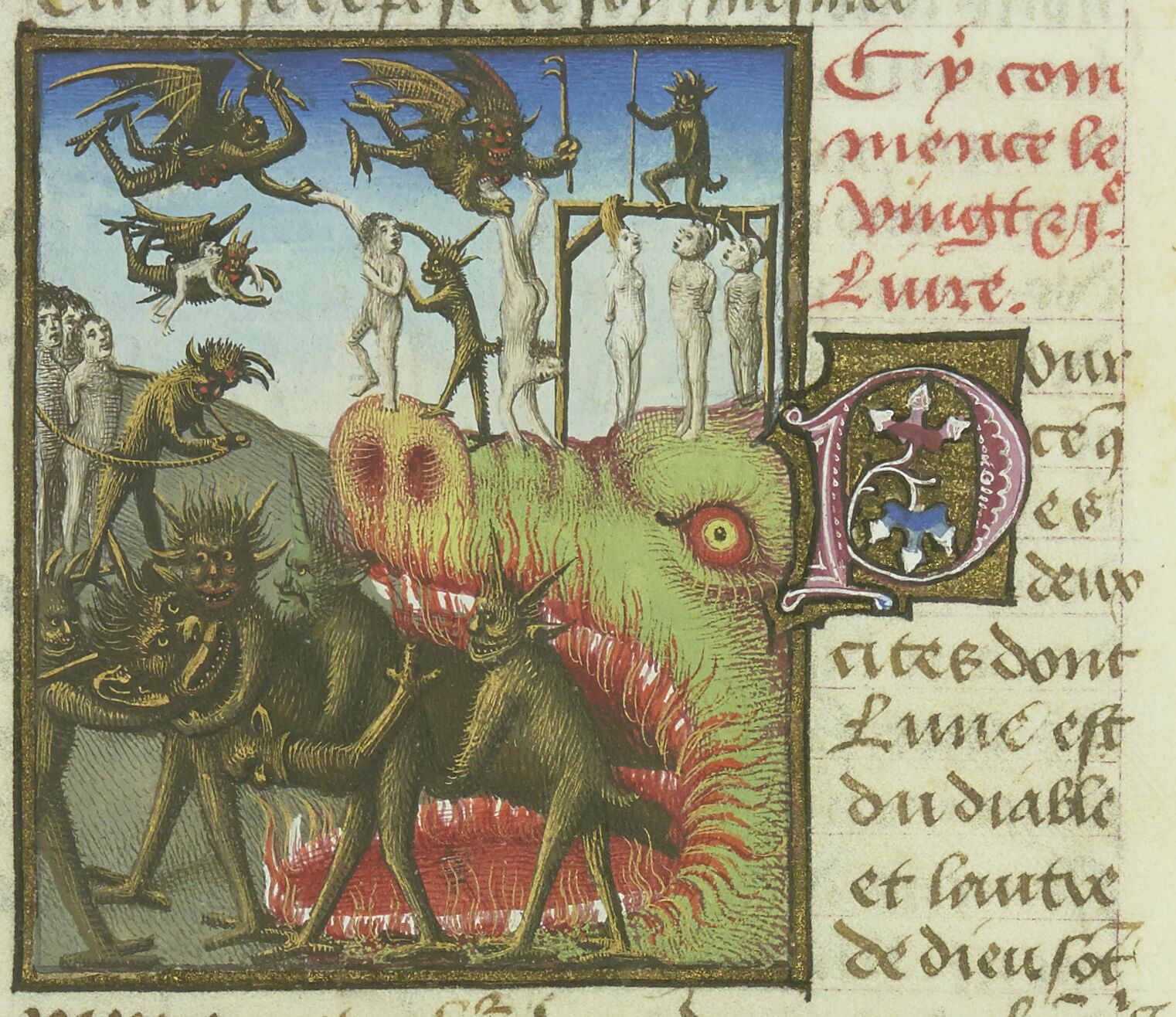This detailed image appears to be an older, animated drawing with a vintage, possibly medieval style. The main feature on the left is a vertical rectangle framed in a brown metal-like border. Inside, a fantastical, ghastly scene unfolds. The central focus is a large greenish monster with sharp white teeth and a vividly red tongue, spewing red fuzz and smaller brown, horned creatures from its mouth. There are several smaller, winged green monsters flying around, as well as monkey-like creatures with spiked hair and horns, some of which are carrying a possibly injured comrade. 

A notable part of this scene is three white human-like figures hanging from a wooden stand in the upper right corner, seemingly bandaged or naked, with some tied by their hair. Below and to the right of this grisly tableau, there's a pig-like dog or boar creature with flames emanating from its open mouth. 

On the right side of the image, there is a light brown, beige background with foreign text. The text includes red print at the top and green print in the middle and at the bottom, with a logo above that – possibly a stylized "P" or "O" adorned with blue and purple flowers. The language is not English and resembles our alphabet letters, suggesting it might be an older script akin to Latin. This detailed depiction, rich with varied colors like green, red, yellow, and black, conveys a nightmarish fantasy world.